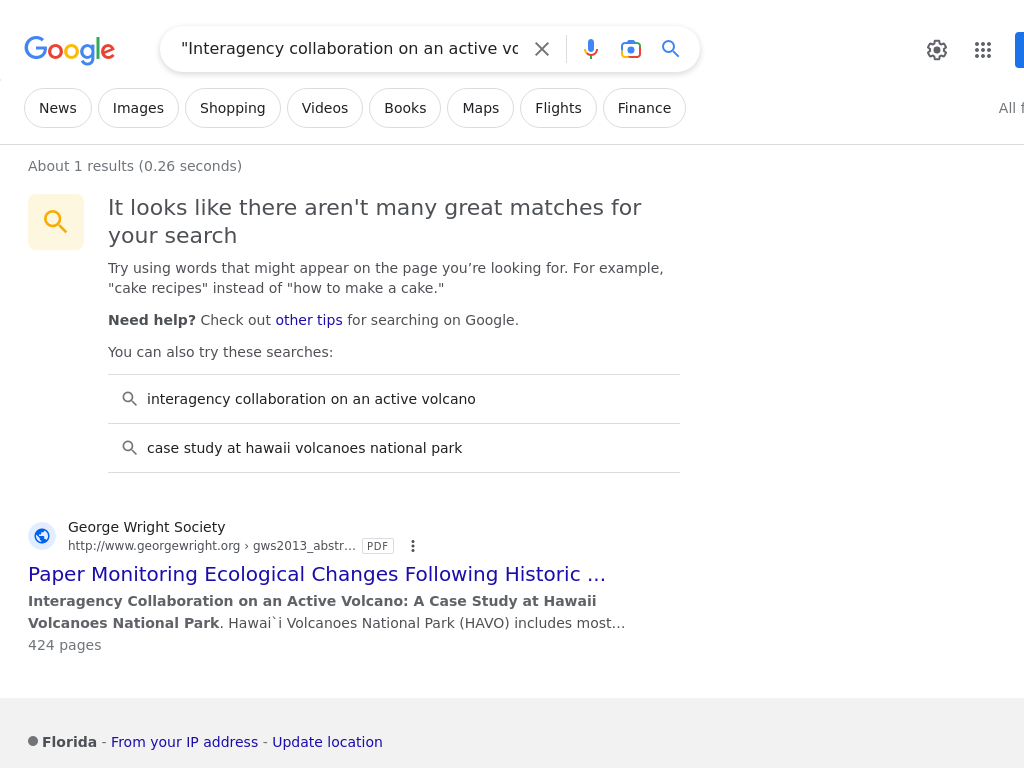The image is a detailed screenshot of a Google search results page with a clean, white background. At the top, the iconic "Google" logo is displayed in its standard multicolored format. Below the logo is a search bar containing the partial search query, enclosed in quotation marks: "interagency collaboration on an active VO..." The bar also includes an 'X' to clear the search, a microphone icon for voice search, a camera icon for image search, and a magnifying glass icon to initiate the search.

To the right of the search bar, there's a gear icon representing settings and a 3x3 dot grid icon, likely for accessing a Google Apps menu. Below this is a horizontal navigation menu with categories including 'All,' 'News,' 'Images,' 'Shopping,' 'Videos,' 'Books,' 'Maps,' 'Flights,' and 'Finance.'

A separator line indicates that there is only one search result, displayed in approximately 0.26 seconds. A yellow search icon is accompanied by a message stating, "It looks like there aren’t many great matches for your search. Try using words that might appear on the page you’re looking for, e.g., 'cake recipes' instead of 'how to make a cake.'" There is a suggestion for additional help with a clickable link to check out more tips for searching on Google.

The page then offers an alternate search query: "interagency collaboration on an active volcano: case study at Hawaii Volcanoes National Park." The solitary search result comes from the George Wright Society's website (www.georgewright.org) and is titled "Monitoring Ecological Changes Following Historic..." It features a preview text: "Interagency collaboration on an active volcano: a case study at Hawaii Volcanoes National Park (HAVO) includes most..."

At the bottom of the page, there is a light gray bar displaying the user's location as "Florida," along with two links: one indicating "from your IP address" and another for "update location."